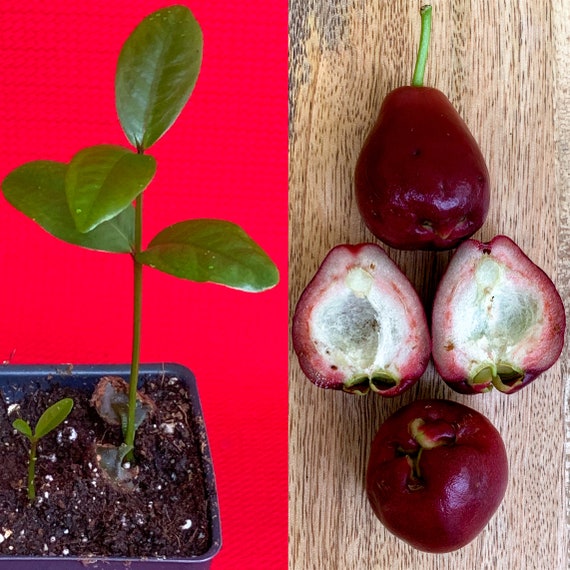The photograph features a side-by-side composition. On the left, set against a vibrant red background, is a small black pot filled with soil. From the soil, a young plant has sprouted with two green stems, each bearing medium-sized, glossy leaves. One stem is slightly taller than the other. The right side of the image displays three pieces of fruit resting on a light brown wooden surface. The fruits, which resemble pomegranates, include two whole fruits with green stems and one fruit cut in half. The outer skin of the fruit is dark red, while the inside reveals a white, fuzzy texture with pinkish flesh near the skin. The seeds are visible at the top of the sliced fruit, completing the detailed depiction.